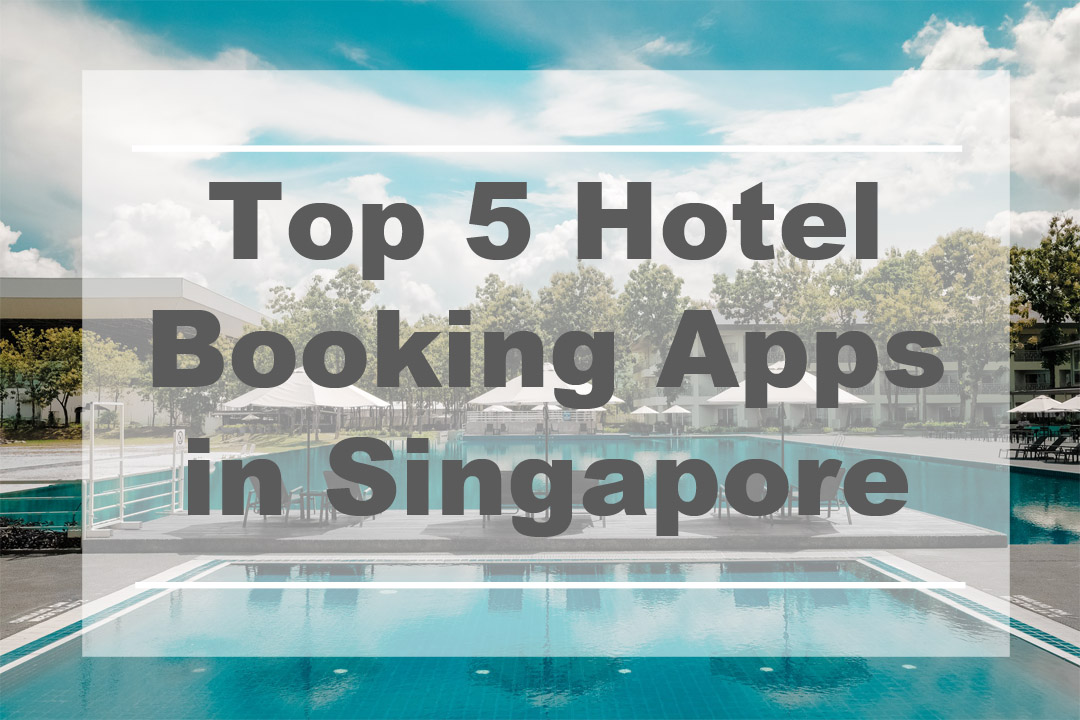A screenshot from an unidentified webpage showcases a serene poolside setting dominated by a shimmering turquoise swimming pool. Surrounding the pool are several white umbrellas, with three prominently positioned in the center of the image. These central umbrellas are mirrored perfectly in the clear pool water, enhancing the tranquil atmosphere. In the background, an array of lush trees stretches across the scene, accompanied by a partial view of a building on the left. Scattered pool furniture adds to the inviting ambiance. The sky overhead is a deep, vibrant blue, dotted with numerous large, white clouds. Overlaying the center of the image, a transparent white square features black text reading, "Top 5 Hotel Booking Apps in Singapore," flanked by thin white horizontal lines above and below the text. The image is devoid of people, animals, birds, automobiles, and bicycles, focusing purely on the picturesque, tranquil poolside environment.